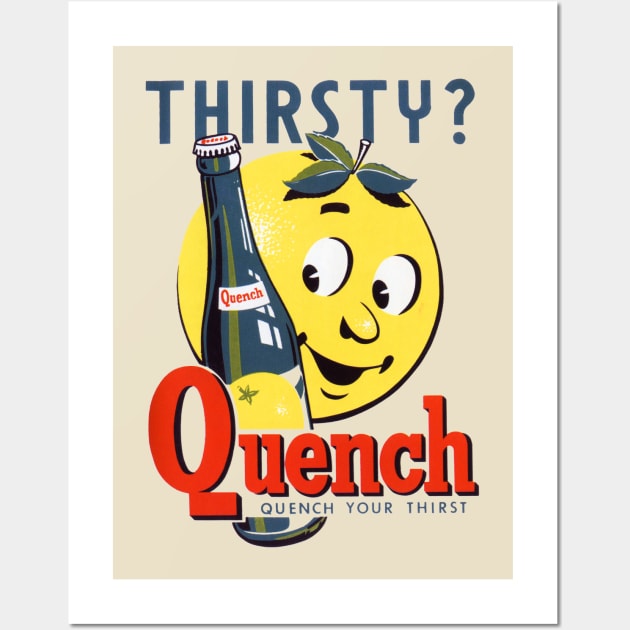This image is a retro-style advertising poster for a soda called Quench, displayed on a white-framed, tan background. At the top, "THIRSTY?" is printed in large, dark teal/blue font. Below it stands a large, cheerful cartoon lemon, bright yellow with three green leaves on its head resembling hair. The lemon has a human-like face, smiling and looking at a glass bottle of Quench soda. The bottle is dark blue-green with a prominently featured yellow lemon on its label. The word "QUENCH" is written in bold orange/red letters across the bottle, which also sports a white cap. At the bottom of the poster, the text "QUENCH YOUR THIRST" is displayed, reinforcing the advertisement's message.